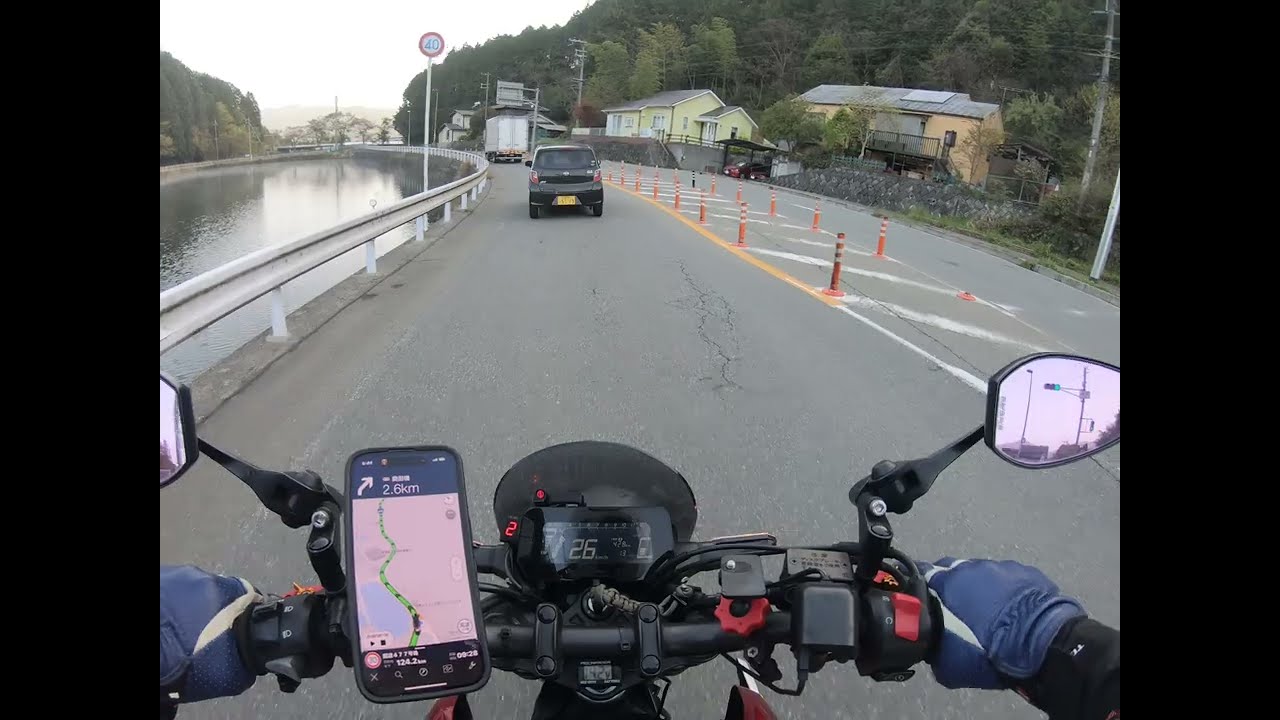The photograph, taken from the point of view of a cyclist on a motorcycle, showcases a detailed, dynamic scene. The image, slightly wider than it is tall, is framed by wide black vertical bars on the left and right. Centered in the lower portion, the motorcyclist's hands grip the handlebars, adorned in dark navy blue gloves with lighter gray accents between the thumb and index finger. The motorcycle is also partly visible, including a digital speedometer displaying "26 km/h" and a mounted cell phone to the left, which shows a GPS screen indicating a turn in 2.6 kilometers with a wavy, green path.

The road is a one-lane asphalt stretch, with a white railing that runs along the left side. Beyond the railing lies a serene lake, reflecting a predominantly overcast sky with some white clouds. In the top left, the sky transitions from white to a cloudy texture. The road curves to the left and is bordered by gentle hills and lush green trees. Further ahead, a black car with a yellow license plate and a white delivery truck lead the way, following the bend.

On the right side of the image, orange traffic barriers with white stripes mark the road’s edge, and there are white diagonal lines painted on the road's surface. Buildings populate the background: a pale yellow house and a lime-green building partially obscured by foliage can be seen against the backdrop of hilly terrain covered with trees. Power lines cross through the background, adding to the sense of a rural yet developed landscape. The motorcycle's mirrors reflect snippets of the scene, with the left mirror showing only part of itself and the right mirror reflecting the pink-tinged sky.